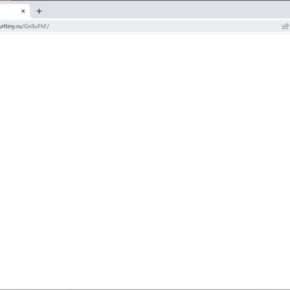The image captures a minimalist web page with an almost entirely blank layout. The predominant colors are muted shades of gray and white, giving the webpage a clean and uncluttered appearance. The address bar at the top contains some partially visible and illegible text, suggesting that a URL is being typed or edited but is not fully displayed. The vast expanse of empty space emphasizes the simplicity of the design and leaves room for further content to be added.